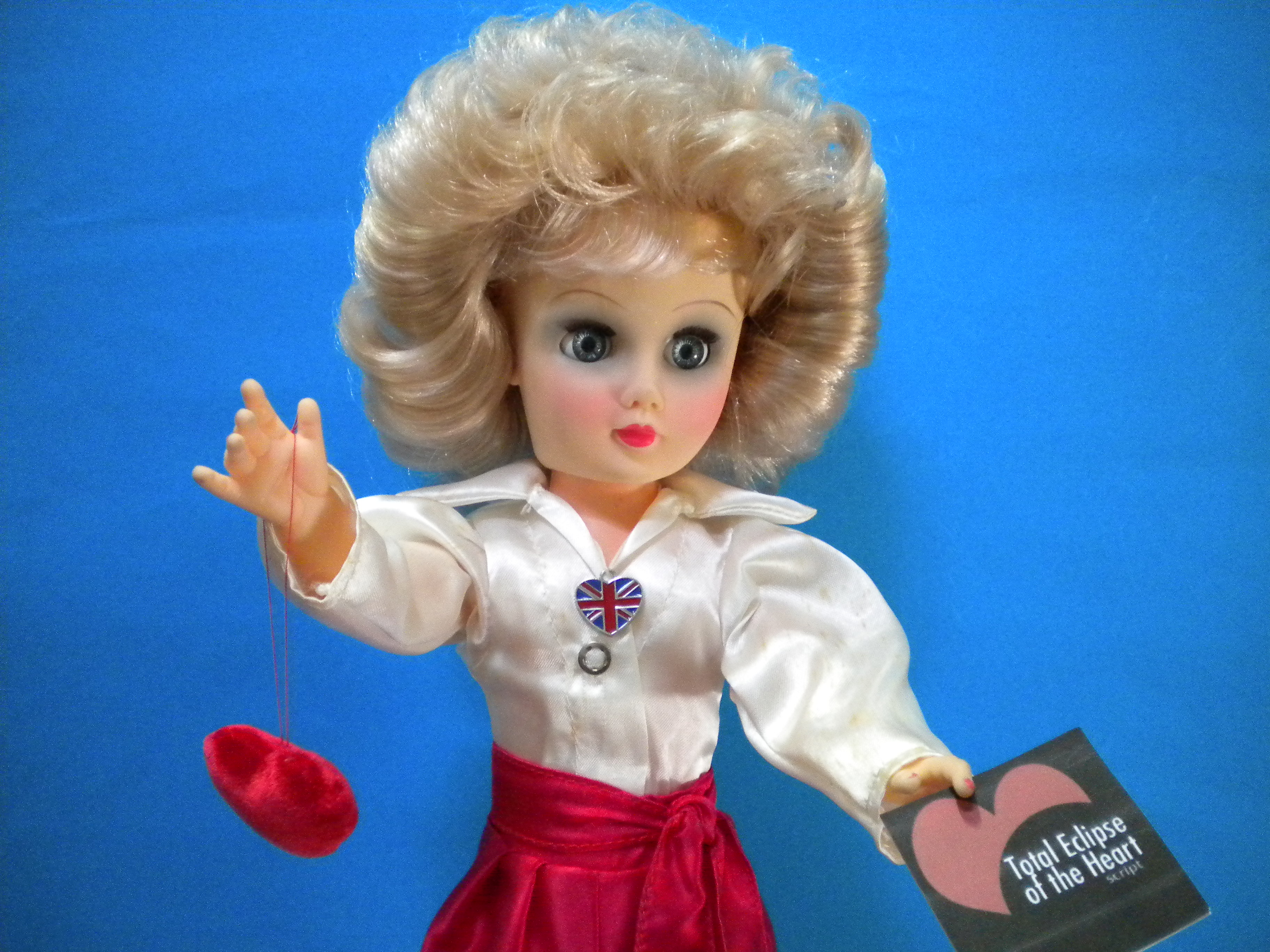The image depicts a commemorative doll crafted with a unique design. The doll resembles a Barbie but with a larger head and is dressed in a white button-up blouse featuring a small heart pin adorned with the British Union Jack flag on the collar. She is also wearing a red skirt complemented by a red sash around her waist. The doll is of a lighter skin complexion, with teased curly blonde hair and strikingly red lipstick, complete with rosy cheeks and a surprised facial expression.

In her right hand, the doll holds a little plush heart hanging from a red string, and in her left hand, she displays a black and red script that reads "Total Eclipse of the Heart" in white letters, partially decorated with a pink heart. The background of the image is a dark sky blue, providing a clear and vivid setting for the doll. The overall quality of the image is very clear, enhancing the visibility of the doll's intricate details. This doll appears to be a tribute to "Total Eclipse of the Heart," potentially linked to the song by Bonnie Raitt.